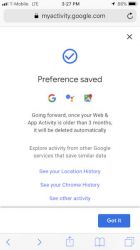In this image, there is a screenshot of the Gokli app page, specifically accessed through the URL "myactivity.gokli.com" visible at the top. Prominently displayed below the URL, there is a blue and white circle featuring a blue tick mark inside, accompanied by the text "Preference saved" underneath.

There are three distinctive icons below this message: 
1. The colorful "G" for Gokli, rendered in red, yellow, green, and blue.
2. An icon representing the Gokli Assistant, shown as four circles colored yellow, green, blue, and red.
3. The recognizable Gokli Maps icon.

Toward the bottom of the page, there's a section labeled "More iOS app activity," although the text is somewhat blurry and hard to decipher clearly. On the bottom right, there is a blue button labeled "Got it."

Further down, three blue-colored options are listed:
1. "See your location history" at the top in blue text.
2. "See your Chrome history" in the middle, also in blue text.
3. "See and activate" at the bottom in blue text.

The rest of the text on the page is primarily written in black, contrasting with the blue elements.